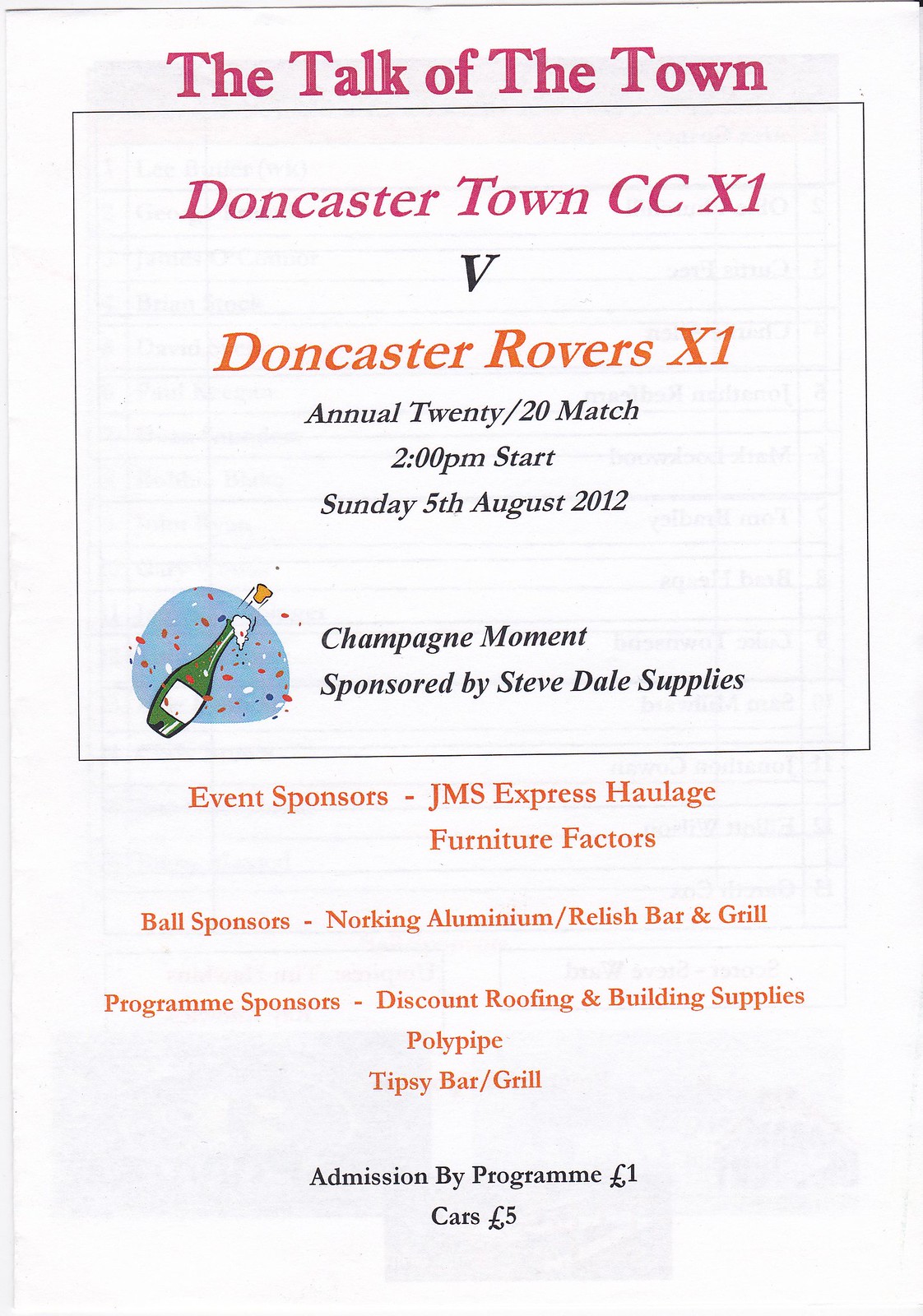The image features a white background with prominent red letters at the top stating "The talk of the town." Below, a thin black rectangle encloses the text "Doncaster Town CCX1," followed by a centrally positioned black "V" and "Doncaster Rovers X1" in lighter red or orange letters. Underneath, smaller black letters announce the "Annual 20/20 Match" with a 2 p.m. start on Sunday, 5th August 2012. In the bottom left corner, there’s an image of a green champagne bottle with a white label, surrounded by a blue circle with multicolored confetti. Adjacent to the image, in small letters, it reads "Champagne Moment" and "Sponsored by Steve Dahl Supplies." Below the black rectangle, in red letters, the event sponsors are listed: JMS Express Haulage, Furniture Factors; ball sponsors: Norking Aluminum, Relish Bar and Grill; program sponsors: Discount Roofing and Building Supplies, Polypipe, Tipsy Bar/Grill. At the very bottom, black letters indicate "Admission by Program: £1, Cars: £5."